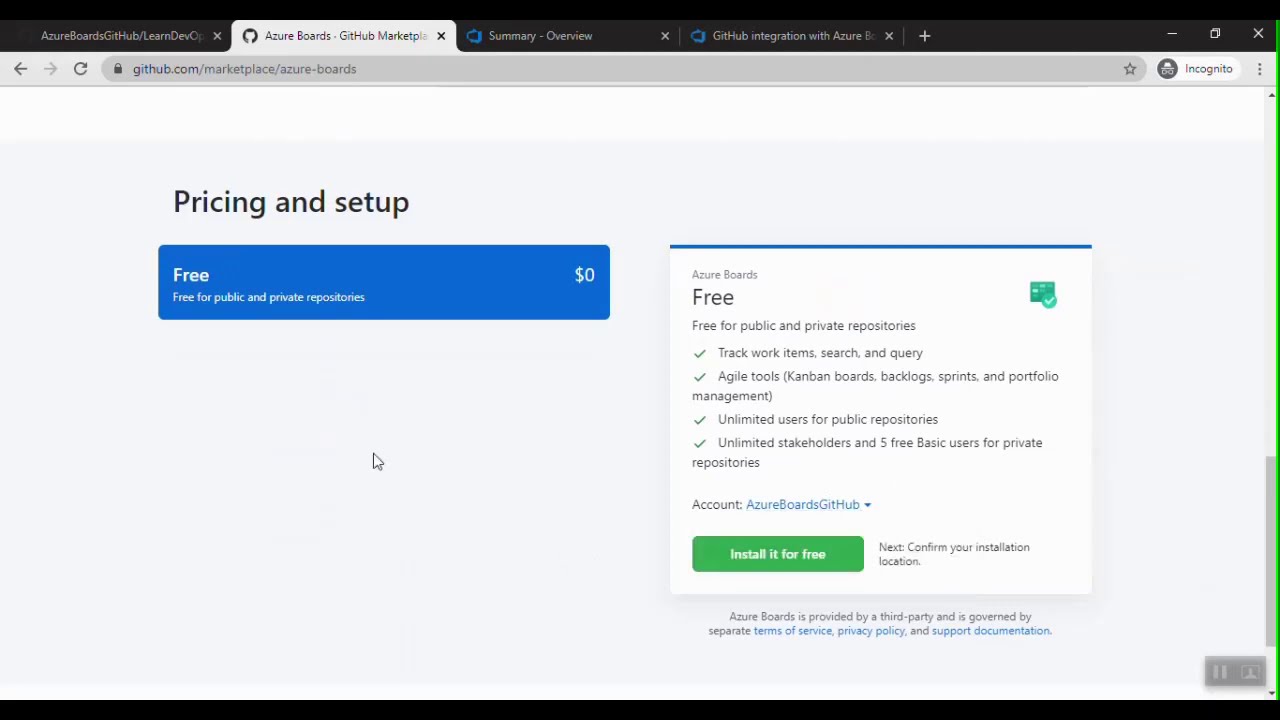A screenshot of a web browser displaying the GitHub Marketplace page for Azure Boards in incognito mode. The browser has four tabs open, with the second tab active, titled "Azure Boards · GitHub Marketplace." The URL in the address bar reads "github.com/marketplace/azure-boards." The typical browser navigation buttons, such as back, forward, and reload, are visible. 

The main content of the page is focused on the Azure Boards offering. On the left sidebar, options for "Pricing" and "Setup" are visible. The central section of the page highlights various features and pricing details within a blue box marked "free," indicating that Azure Boards is free for both public and private repositories. Below this, two options are detailed:

1. **Pricing Plan:** 
   - **Free for Public and Private Repositories** 
   - Cost: $0

2. **Azure Boards Features:** 
   - Track work items, search, and query.
   - Agile tools including Kanban boards, backlogs, sprints, and portfolio management.
   - Unlimited users for public repositories.
   - Unlimited stakeholders and five free basic users for private repositories.

Further down, there is an "Account" section with a dropdown labeled "Azure Boards GitHub" and a green button that says "Install it for free." Adjacent to this button, there's text advising to confirm the installation location. Below this, a note clarifies that Azure Boards is provided by a third party and is subject to separate terms of service, privacy policy, and support documentation.

The page is simple and primarily informative, emphasizing Azure Boards' features, system usage, and installation instructions.